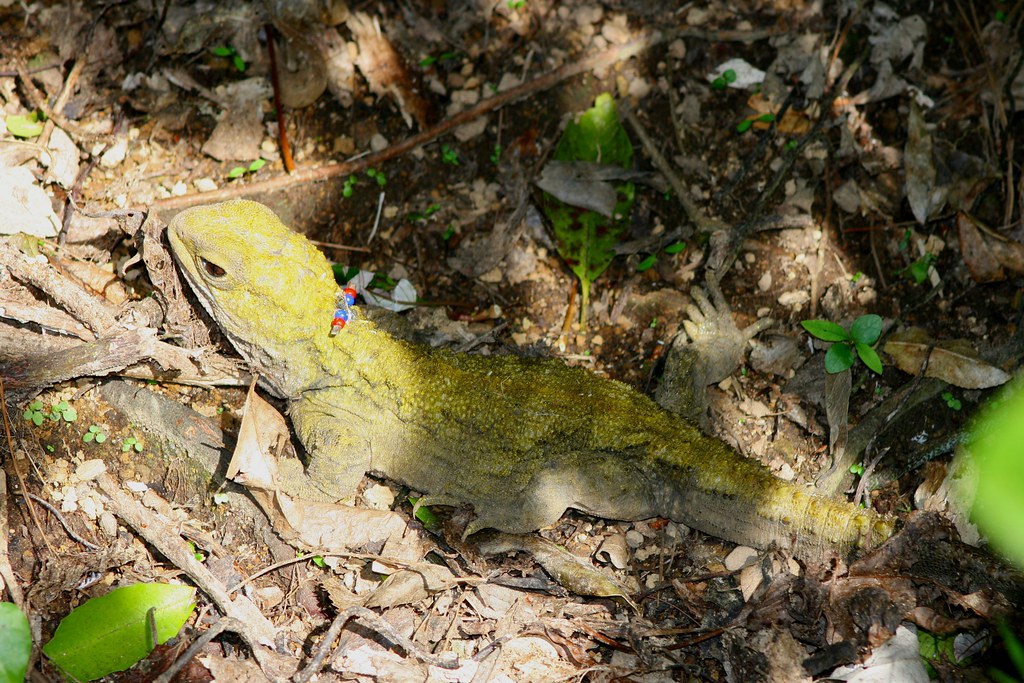The photograph captures a side view of a lizard, likely a gecko or iguana, resting on the ground outdoors amidst a scattered array of natural debris. The lizard’s body features a distinctive mossy green coloration with a scaly texture along its back and tail, blending seamlessly with its surroundings. The rest of its body showcases a spectrum of colors including light brown, tan, and gray, with a notably wrinkly appearance. A close inspection reveals what appears to be a tag, possibly made up of small red and blue beads, situated on the back of its neck. The ground beneath the lizard is strewn with a variety of elements: dry, dead brown leaves, brown branches, bits of dirt, and occasional pockets of bright green, fresh leaves. The composition includes a green leaf prominently in the lower left corner and various sticks, rocks, and weeds, all contributing to the natural, outdoor setting. The lizard’s brown eye gazes out, adding a lifelike detail to the scene, which is rich with texture and natural clutter, painted in earthy tones accented by sporadic greenery.